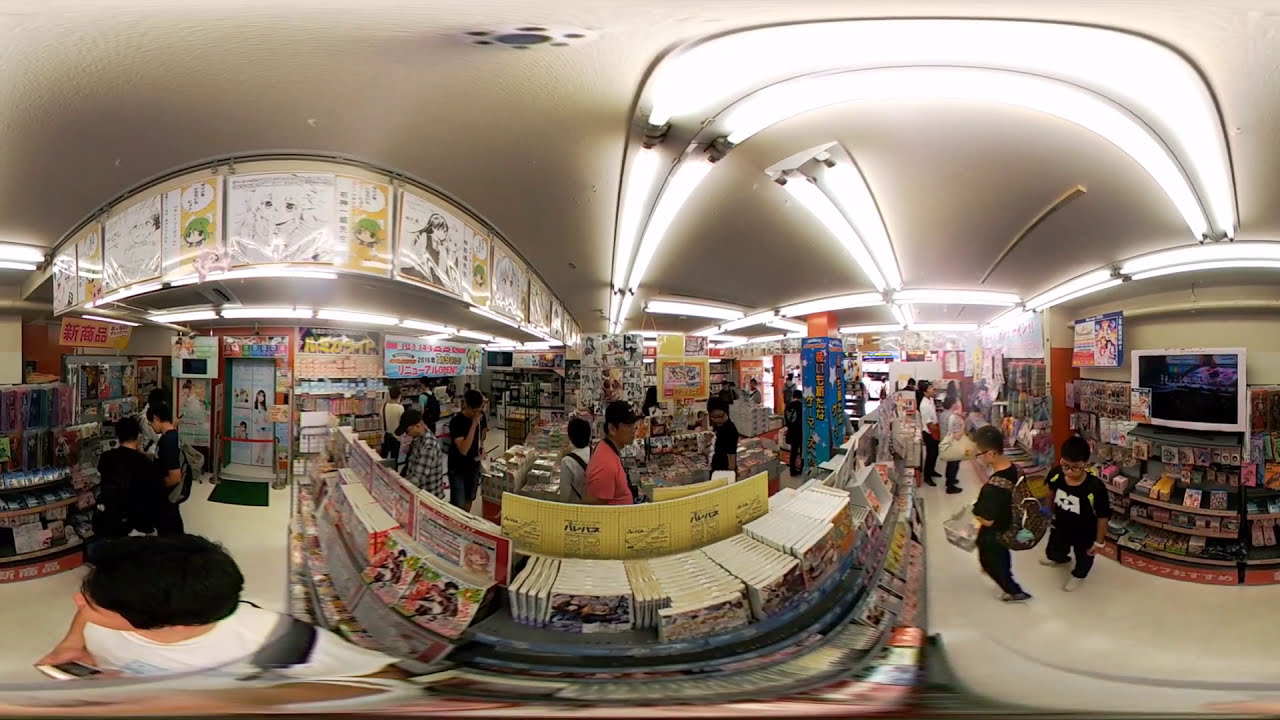This is a fisheye, 360-degree image taken inside an Asian store, possibly located in Japan, China, or Korea, as indicated by the presence of Japanese, Chinese, and Korean lettering throughout. The inside of the store is brightly lit by fluorescent lights, with a stark white floor and ceiling. The photograph, with its characteristic distorted lines, gives a comprehensive view from above, seemingly captured by a man with medium skin and black hair, wearing a white t-shirt and holding his smartphone above his head.

In the immediate foreground are rows of books, possibly comics or DVDs, indicative of extensive reading material available. There's a noticeable presence of packaged food items and various boxes on display. Anime posters and drawings, mostly featuring young anime characters, are prominently hanging from the center to the left side of the ceiling, advertising and explaining store items. An LCD screen on the right side showcases additional products for sale beneath it, with two patrons standing nearby, one holding a shopping basket.

The store has several patrons, predominantly male, some perusing items, others seemingly standing in line. To the bottom left of the image, there's a male patron in a white shirt holding a phone, with two other males positioned behind him. A green floor mat leading into an entrance can be seen right behind these individuals. Various displays, possibly containing candies or food items, are scattered throughout the store, emphasizing the diverse range of products offered.